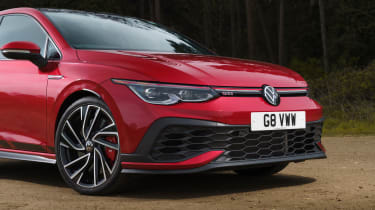This detailed image captures the front view of a sporty, red Volkswagen sedan, partially cropped just behind the side view mirrors. The car's striking appearance is accentuated by black and silver rims, chrome hubcaps, and a black woven grille adorned with the iconic VW logo. The narrow, slanted headlights enhance its sleek design, while the white license plate reads G8VWW. The windshield and the side window reflect the bright sunlight and surrounding trees. The car is positioned on a simple dirt road, contrasting with the dense backdrop of tall trees and dark, lush bushes, suggesting it is parked in a wooded area.